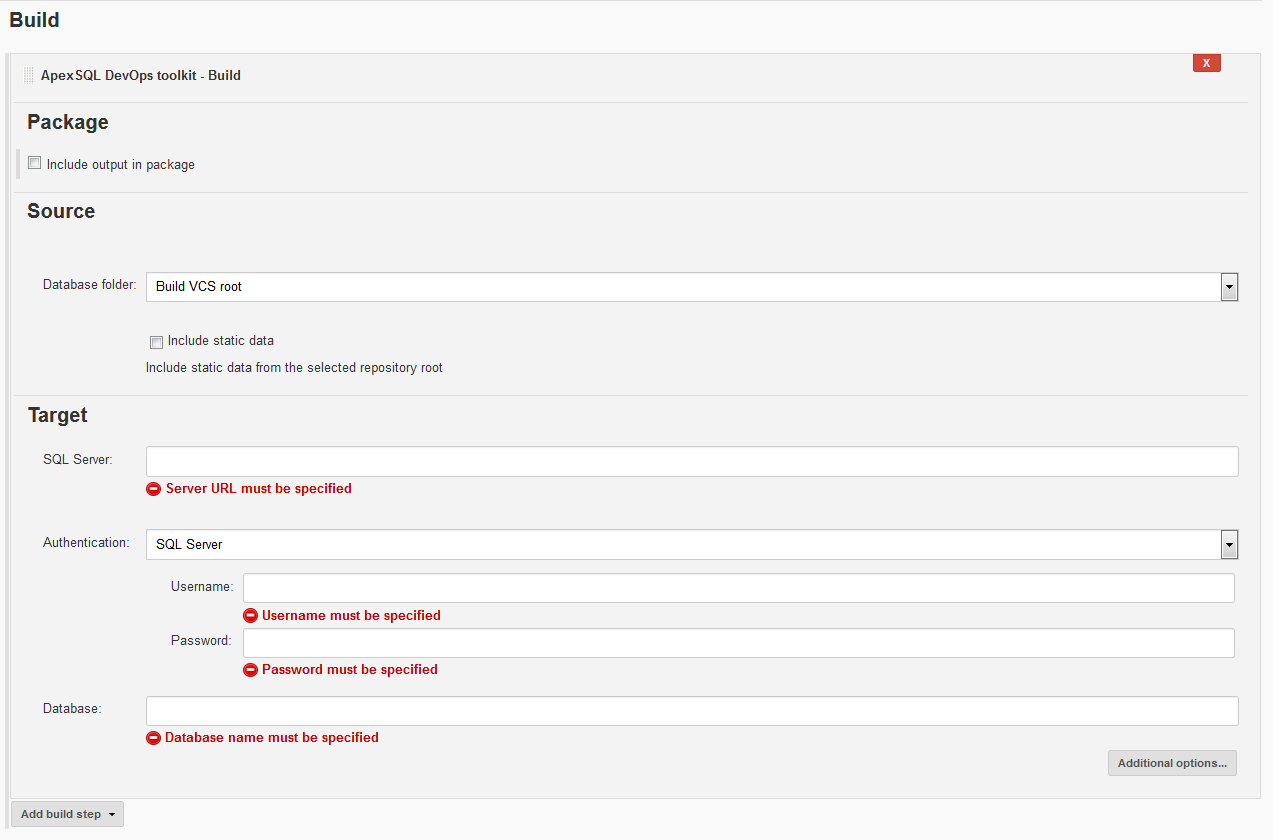This image is a screenshot from a webpage, specifically from a section titled "Build" displayed prominently at the top in black print. The surrounding background of the entire section is light gray. Just below the title, the text "Apex SQL DevOps Toolkit" is clearly visible, followed by another "Build" label.

Further down, a heading labeled "Package" is visible, with an option that reads "Include Output in Package." Progressing through the interface, there is a "Source" section which lists details such as "Database Folder" and "Build VCS Root."

Lower down is the "Target" section, focusing on SQL Server configuration. Within this section, several mandatory fields are highlighted in red ink to indicate incomplete requirements. These include:

- **Server URL:** Marked with a warning stating "Server URL Must Be Specified."
- **Username:** Highlighted with "Username Must Be Specified."
- **Password:** Labeled with "Password Must Be Specified."
- **Database:** Indicating "Database Name Must Be Specified" in red ink.

Each of these fields has a red negative indicator, denoting the necessity for this information to move forward.